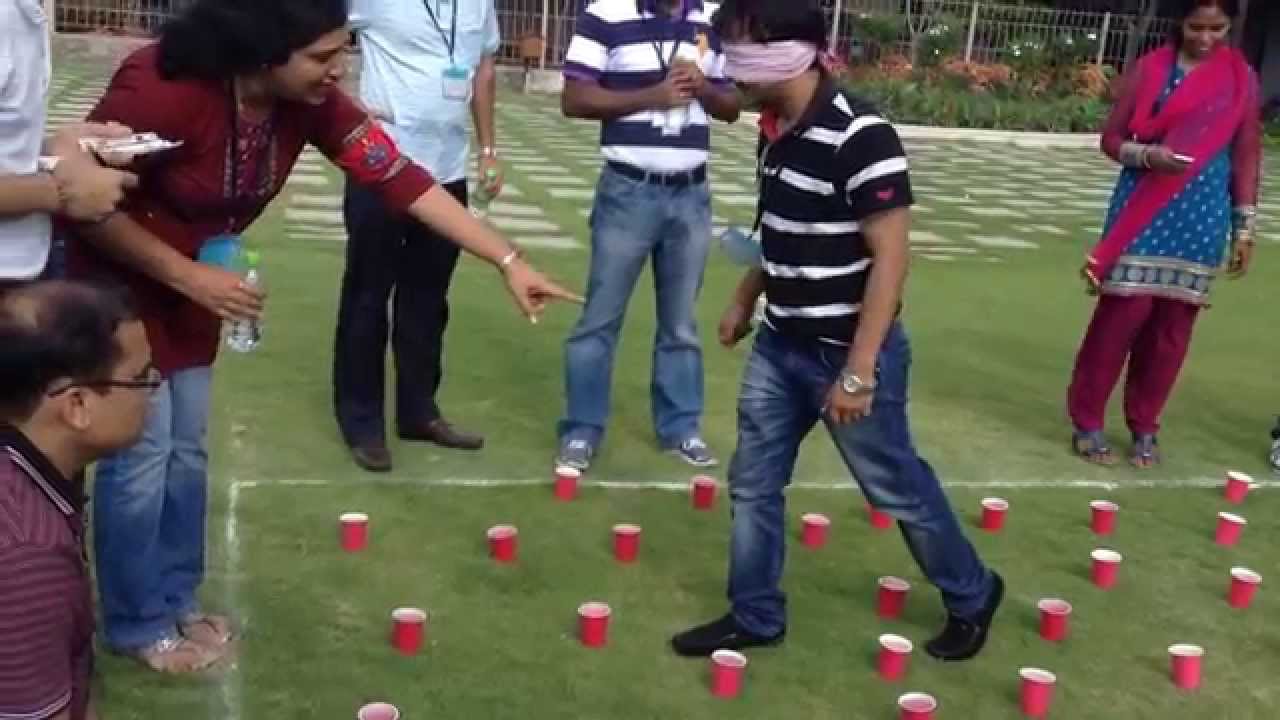In the photograph taken outdoors on a grass field, a man in a black and white striped shirt and jeans is navigating through a grid of red plastic cups while blindfolded. The cups are arranged within a chalk-outlined area on the grass, resembling a minefield he attempts to traverse without knocking over any cups. Surrounding him are groups of onlookers; a woman to the left, wearing a red shirt and holding a water bottle, points at the cups, possibly giving instructions. Another woman near the top right, dressed in traditional Indian attire and with a scarf around her shoulders, smiles as she looks down at her phone. Almost all individuals are wearing lanyards, suggesting they are part of an organized event. The overcast sky casts a dull light over the scene, indicating a cloudy day.